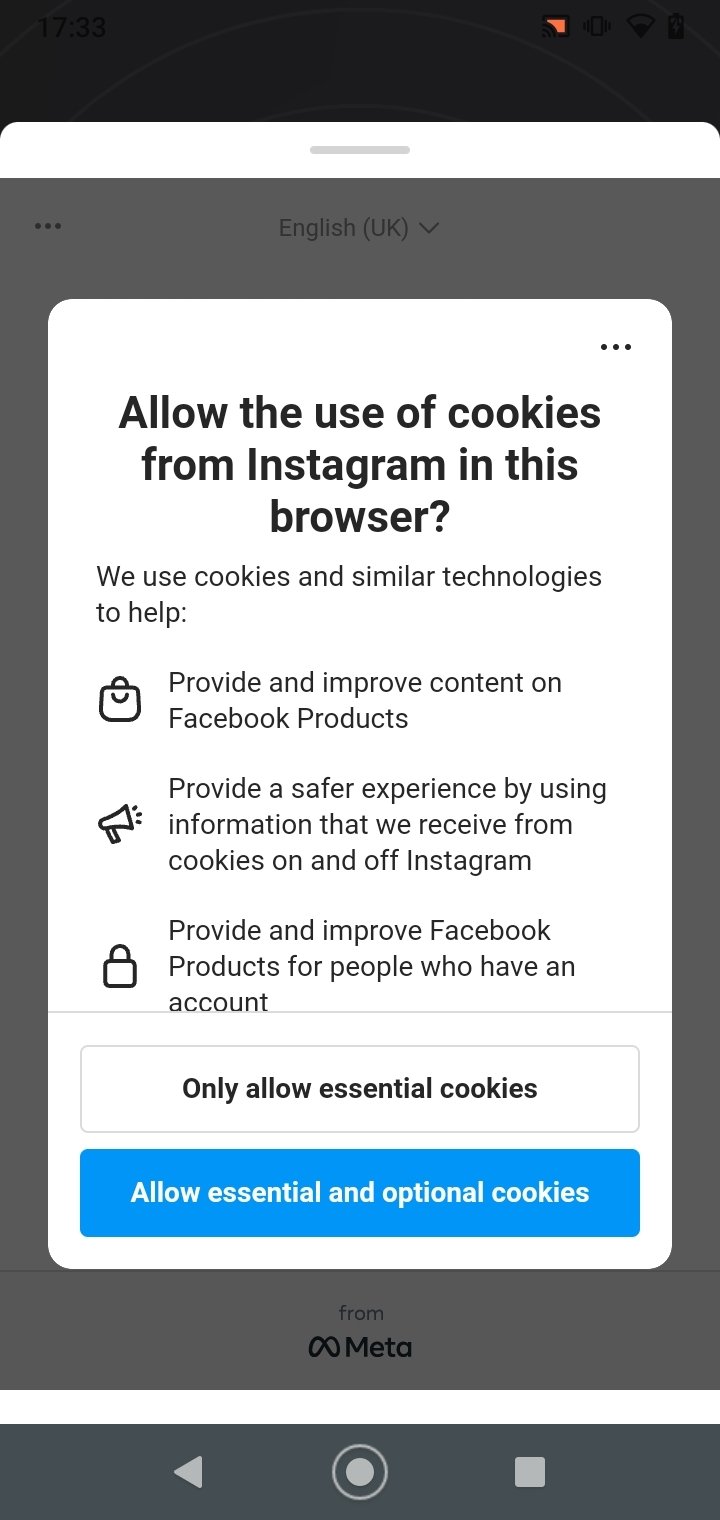In this image, we see a screenshot taken from a phone, depicting a pop-up notification from Instagram regarding cookie usage. The notification is contained within a white square overlaying the blurred, greyed-out background. The message in the pop-up reads, "Allow the use of cookies from Instagram in this browser. We use cookies and similar technology to help provide and improve content on Facebook products, provide a safer experience by using information that we receive from cookies on Instagram, provide and improve Facebook products." 

Below the message, there are two clickable options: "Only allow essential cookies" and a blue button labeled "Allow essential and optional cookies," offering choices for cookie preferences. At the top of the pop-up, there are three vertical dots suggesting additional options or settings. 

In the blurred background, partially visible text reads "English (UK)" above its own set of three vertical dots, indicating language settings. At the bottom of the image, the word "Meta" is displayed, indicating the overarching company brand. Additionally, there appears to be a recording interface with a square icon, suggesting a stop button, and a play button, indicating the potential for media control or playback.